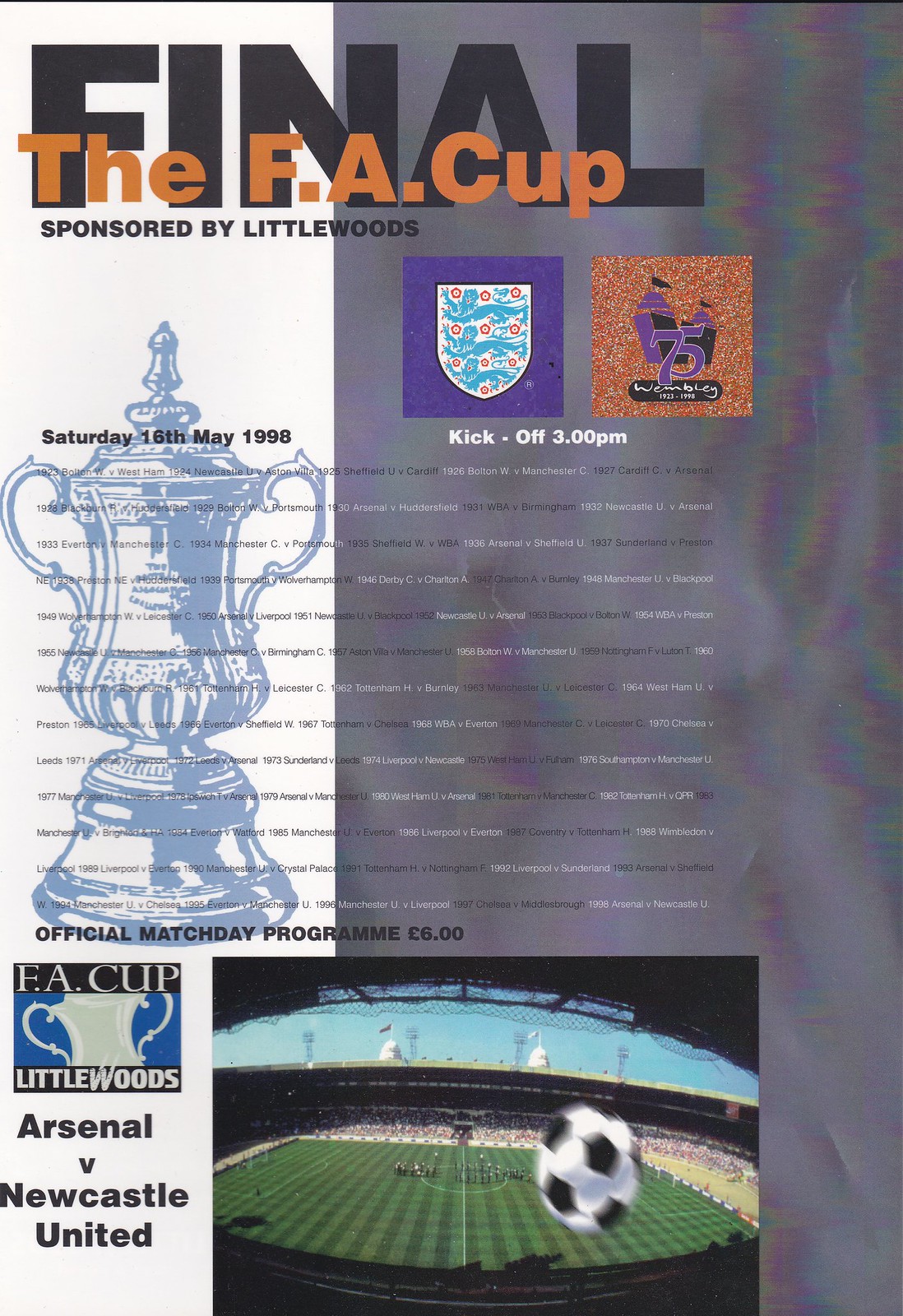The cover for the official matchday program of the 1998 FA Cup Final, sponsored by Littlewoods, prominently features detailed elements to captivate soccer enthusiasts. Dominating the left side of the cover, a translucent blue and white trophy overlayed with the date "Saturday 16th May 1998" in black text and the price "official matchday program six pounds" commands attention. Below it, set against a blue background, there’s a silver trophy illustration accompanied by the prominent "FA Cup Littlewoods" branding and the match headline "Arsenal vs. Newcastle United."

To the right, the background transitions to a textured gray with distinct graphic elements, including a purple rectangle adorned with a 75-year commemorative blue and red shield. The bold header reads "FINAL" in all caps, with "The FA Cup" in overlapping orange text and "sponsored by Littlewoods" below in black. Positioned in an eye-catching spot, the kickoff time "3 p.m." is displayed in white.

Moving towards the bottom, a vivid photograph captures the dynamic action of a soccer ball surging into a net on a field, framed against the blue sky with an overhead view of seating and netting. The program also highlights historical context with a mention of "Wembley 1923 to 1998" and lists notable matchups from Bolton Wanderers vs. West Ham in 1923 to Arsenal vs. Newcastle United in 1998, encapsulating 75 years of FA Cup history.